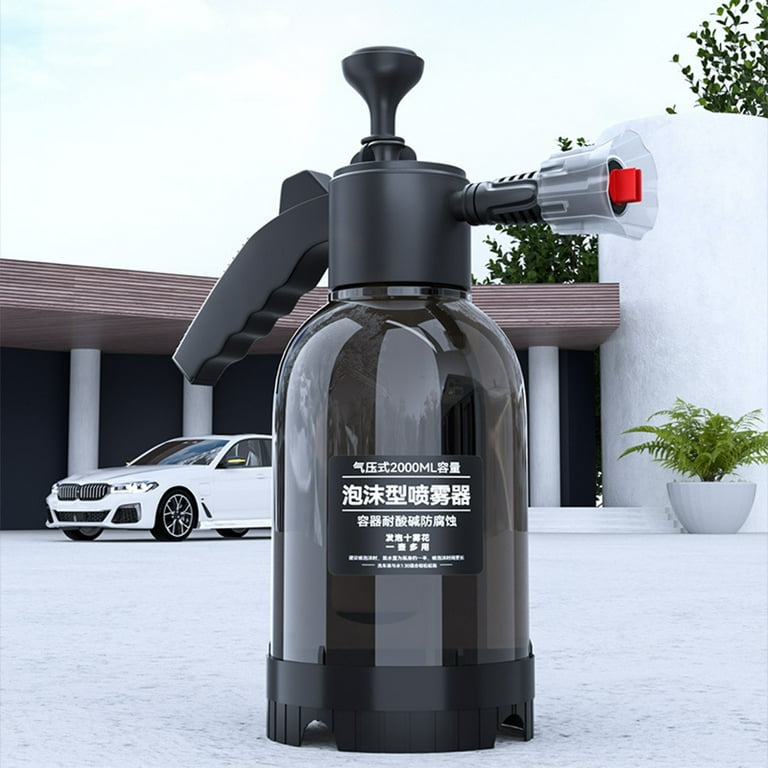The image captures a vertical, rectangular photo featuring a black spray bottle with a red nozzle tip and a label adorned with Asian characters, indicating a capacity of 2,000 milliliters. The bottle, equipped with a trigger-handle mechanism, is set against a backdrop that includes a white car, possibly a BMW, Jaguar, or Saab, positioned on a white concrete surface. In the background, there is a building with white pillars and a black wall, as well as a large white planter containing a green fern-like plant under a sky that is predominantly blue with some white areas.